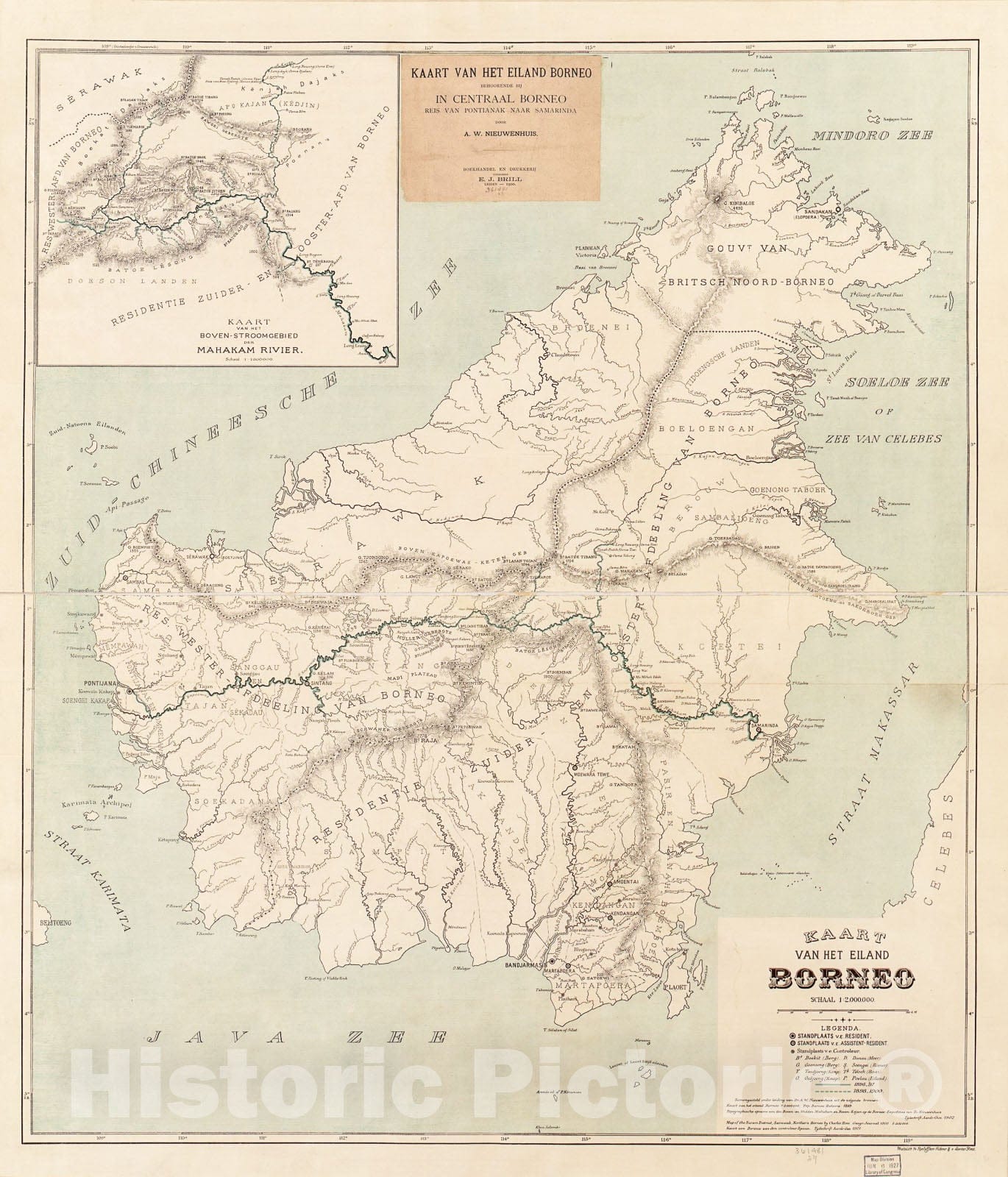This image depicts a detailed historic map of the island of Borneo. The map features a beige and tan background with a black-outlined green landmass. At the top, the title reads "KART VAN HET EILAND BORNEO", indicating the map is labeled in Dutch. Additional small text is scattered across the map, some of which is too small to decipher. Notable Dutch names on the map include the Mindoro Sea, Zuid Chinese Zee (South China Sea), and Java Zee (Java Sea). The lower part of the map bears a watermark that says "Historic Pictoric". To the left of the title, there is a black and white inset showing another landmass, not identical to the main image. The map's topography is detailed with lines depicting landscape features, roads, rivers, and tributaries. The main image of Borneo is shaped somewhat like a squid, wider at the bottom left, and tapering towards the top right. The lower right of the map also includes a legend and shows parts of the Celebes Islands and the Makassar Strait (Strait van Makassar). The author's name appears at the bottom right as A.W. Nieuwhenheuer alongside more small, nearly unreadable text.